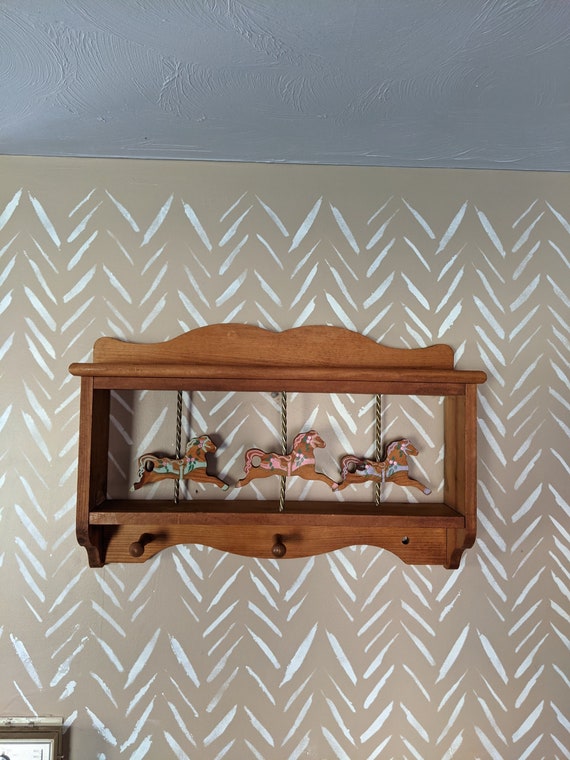This vertically oriented, realistic photograph captures a dark brown wooden coat rack prominently displayed against a tan wall adorned with white V-shaped brush strokes. The wall design resembles vertical, incomplete triangles. Suspended in the coat rack’s central section, three carousel horses are attached via metal rods, each uniquely adorned with colorful saddles: one blue, one pink, and one green. At the bottom of the coat rack, there are two hanging knobs on the left, while a missing third knob on the right leaves a visible hole. The upper part of the image shows a slate-colored ceiling, and in the bottom right corner, a portion of a brown picture frame with a white mat is visible. The overall scene suggests a room with a mix of functional and decorative elements.